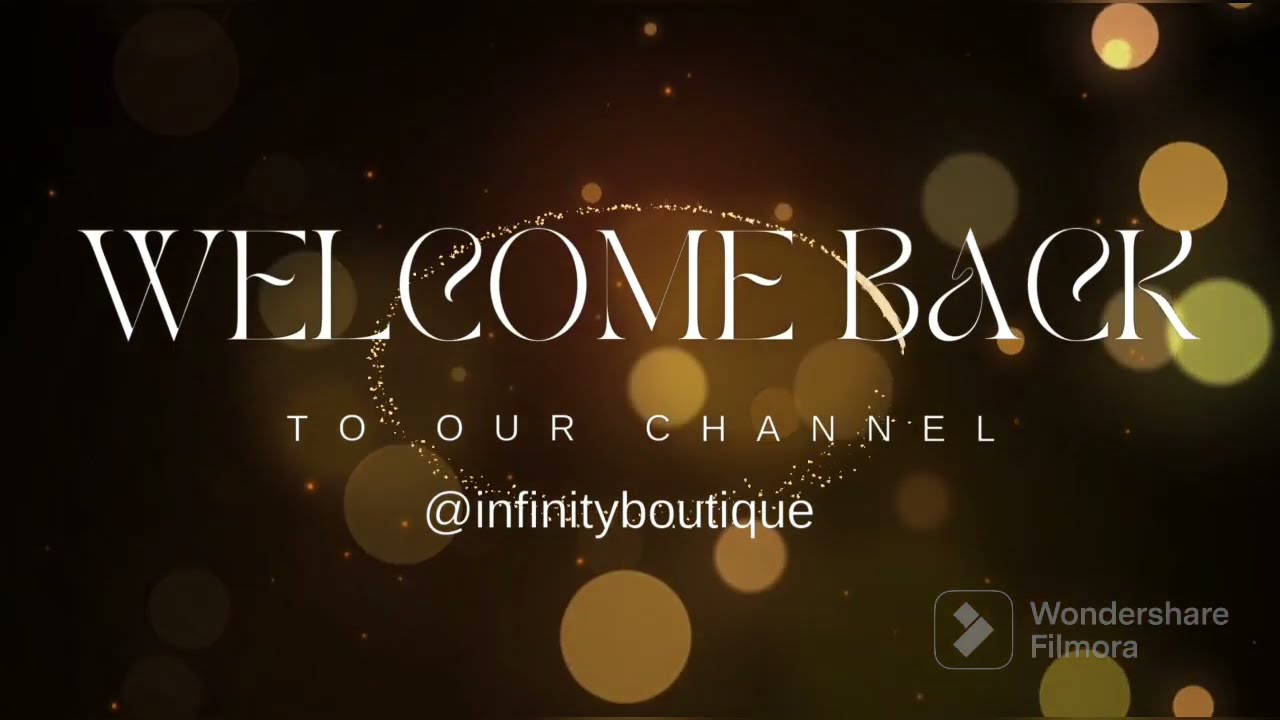The image is a screenshot of a TV screen featuring a graphical design centered around a welcoming message. In bold, white text at the center, three lines read: "Welcome Back," "To Our Channel," and "At Infinity Boutique." The background is primarily dark, almost black, with various circles scattered throughout. These circles range in color from green and gray to orange-ish brown and tan, resembling out-of-focus light sources. These circles vary in size, with the smallest being tiny and the largest about the size of a penny. Additionally, a warm glow radiates near the center of the image, enhancing the text. In the bottom right corner, a watermark with the words "Wondershare Filmora" is displayed in off-white font, accompanied by a logo that appears to be an arrow formed by two squares inside a larger square. Behind the central text is a sparkly circle, which appears as an oval from the perspective of the camera, adding to the overall aesthetic.